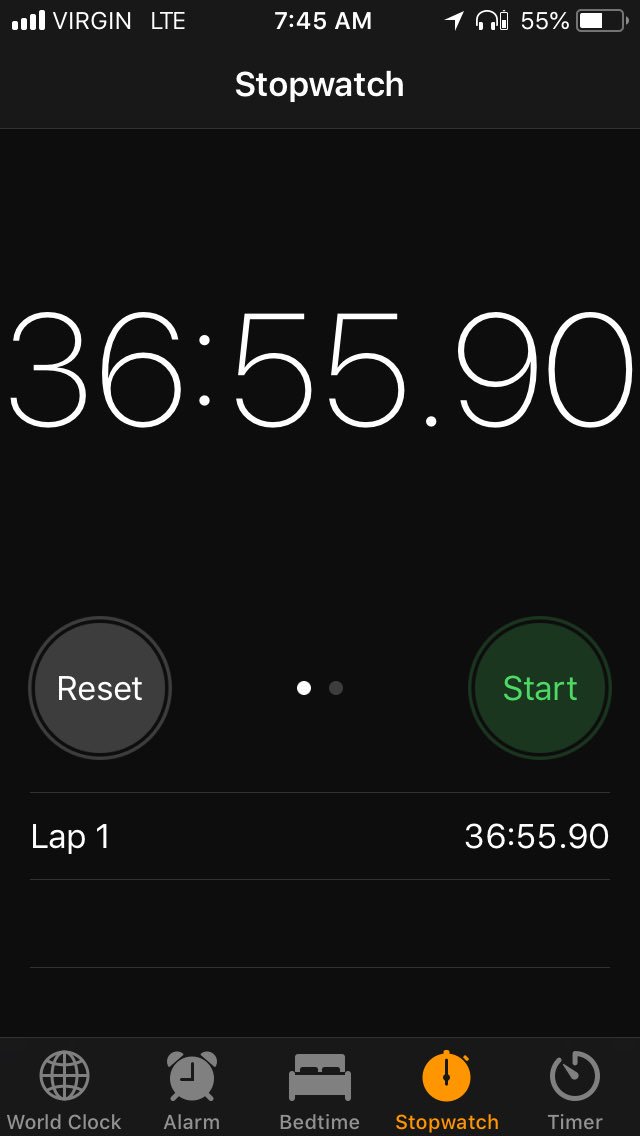The image showcases a mobile device screen featuring a digital stopwatch application against a black background. The top left corner displays the carrier information as "Virgin LTE," accompanied by white signal bars. The current time is shown as 7:45 AM, alongside several icons: the location symbol (a white arrow), headphones, and a battery level indicator at 55%.

Central to the screen is the prominently displayed stopwatch function. The bold numerals "36:55.90" indicate the recorded time, with controls for "Reset" (with a white dot at the center) and "Start" (highlighted in green). Below this is the first lap time, labeled as "Lap 1," showing "36:55.90." 

Subsequently, the bottom section of the screen is an interface for different functionalities of the clock app. These include "World Clock" (with a globe icon), "Alarm" (accompanied by an alarm clock symbol), "Bedtime" (featuring a bed icon), "Stopwatch" (highlighted in orange with a stopwatch icon), and "Timer" (with its corresponding timer icon), all against an entirely black backdrop.